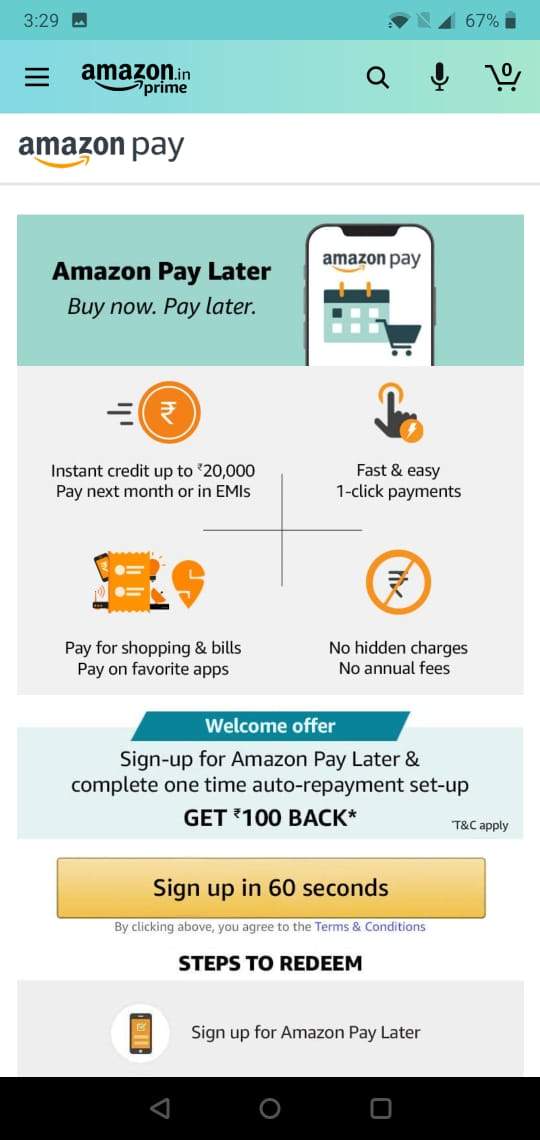Screenshot of an Amazon Pay promotional page on a smartphone taken at 3:29 PM with a 67% battery charge remaining. The screen features a blue border at the top displaying "Amazon.in," along with the Amazon logo and the word "Prime." Beneath that, the heading "Amazon Pay" is prominently displayed, followed by the subheading "Amazon Pay Later: Buy Now, Pay Later."

Central to the screen is an illustration of a smartphone displaying various Amazon Pay related icons: a calendar, a shopping cart, and four additional icons. 

Descriptions of Amazon Pay Later perks are listed below the illustration:
- An icon resembling a coin with the text "Instant Credit up to $20,000, pay next month or in EMIs."
- A finger icon with the text "Fast and Easy One-Click Payments."
- Various icons labeled "Pay for Shopping and Bills," "Pay on Favorite Apps."
- A veto sign stating "No Hidden Charges, No Annual Fees."

At the bottom of the page, a section titled "Welcome Offer" invites users to sign up for Amazon Pay Later and complete a one-time auto-payment setup to receive $100 back, subject to terms and conditions. It emphasizes that the sign-up process takes only 60 seconds, with additional steps for redemption described below.